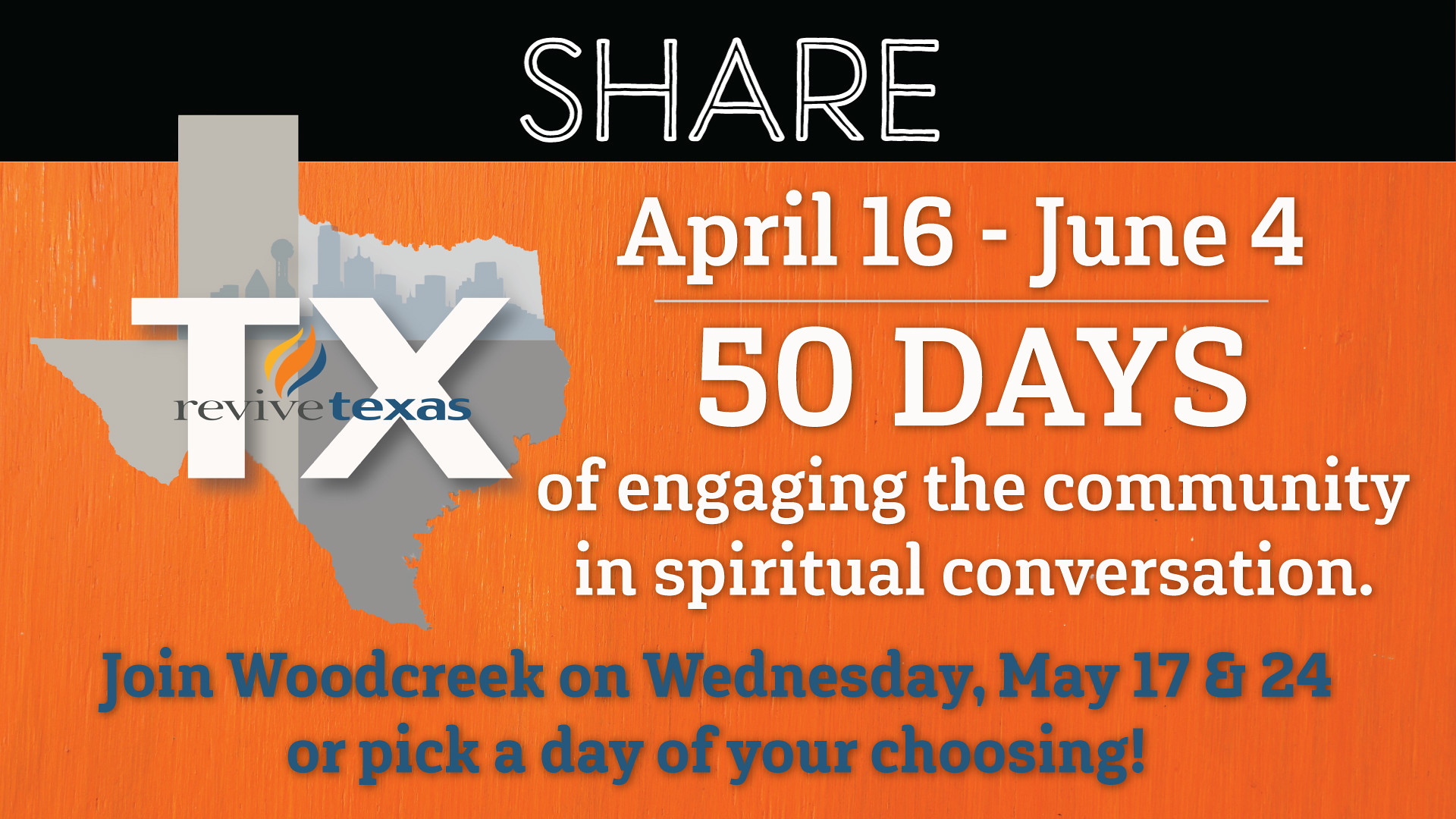This ad blends a sleek design featuring a black strip at the top with the word "SHARE" centered in white, below which lies a textured orange background. On the left side of the orange background is a detailed map silhouette of Texas, overlaid with large "T" and "X" letters and the phrase "Revive Texas" in a smaller font. The ad promotes an event running from April 16th to June 4th, inviting the community to engage in 50 days of spiritual conversation. Further details are provided in white text, specifying dates and event activities. Additionally, in blue text, it encourages participation with "Join Woodcreek on Wednesday, May 17th and 24th, or pick a day of your choosing!" The Texas map logo is distinctively divided into four colors, adding a vibrant touch to this promotional material, which could easily be a newspaper ad, magazine insert, online banner, or a flyer.